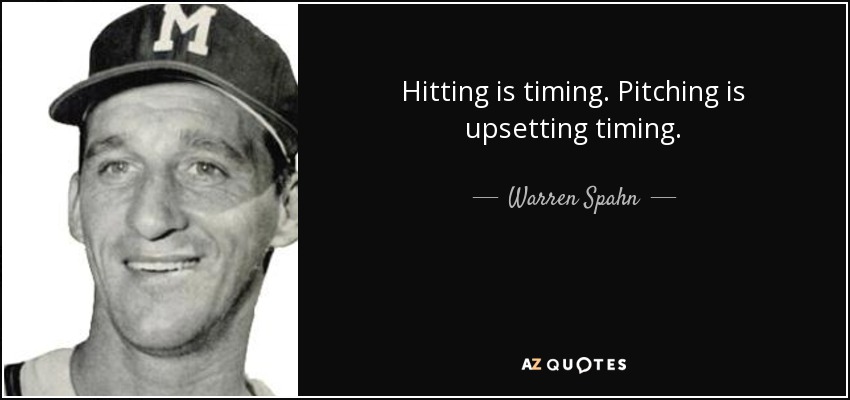The image is a black and white photograph of an older man wearing a dark baseball cap, which features a light-colored capital "M" stitched at the center. He has a warm smile that adds a friendly touch to his face, characterized by slight wrinkles that hint at his age. The image extends from the top of his hat to the bottom of his neck and part of his shoulders.

Adjacent to the man's image, on the right, is a black rectangle with a powerful quote in white text: "Hitting is timing, pitching is upsetting timing." Below this quote, in elegant cursive, is the name "Warren Spahn," flanked by two dashes on either side. At the bottom of this black section, the source "AZ Quotes" is prominently displayed, with the "O" in "Quotes" cleverly replaced by a white speech bubble filled with black. The letter "Z" in "AZ" is highlighted in peach, contrasting with the otherwise white text. The overall background behind the man's picture is white, providing a stark contrast to the black rectangle, making both the image and the text stand out distinctly. This detailed composition likely portrays Warren Spahn, who was a renowned professional baseball player known for his extraordinary pitching skills.